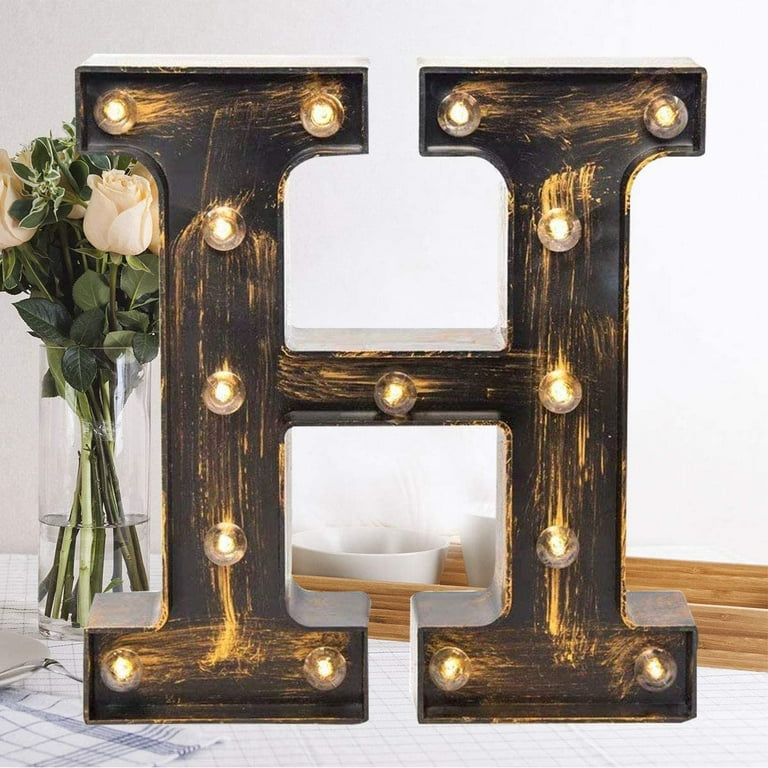The image features a large, decorative letter "H" designed to be a centerpiece for a mantle or table. The "H" has a faux distressed patina, primarily black with distressed elements in a yellowy gold hue, giving it an antique look. It is accented with small, round light bulbs lining the inside, ready to light up. The "H," made of wood and stained in a dark brown, stands about as tall as a long-stemmed rose. This decorative piece is set against a white grid surface and is accompanied by a blue and white plaid hand cloth to its left. In the background, there's a clear vase densely packed with pale peach-colored roses and abundant green leaves, the water level sitting almost halfway up the vase. Additionally, a white ceramic bowl can be seen behind the letter "H," adding to the overall composition.